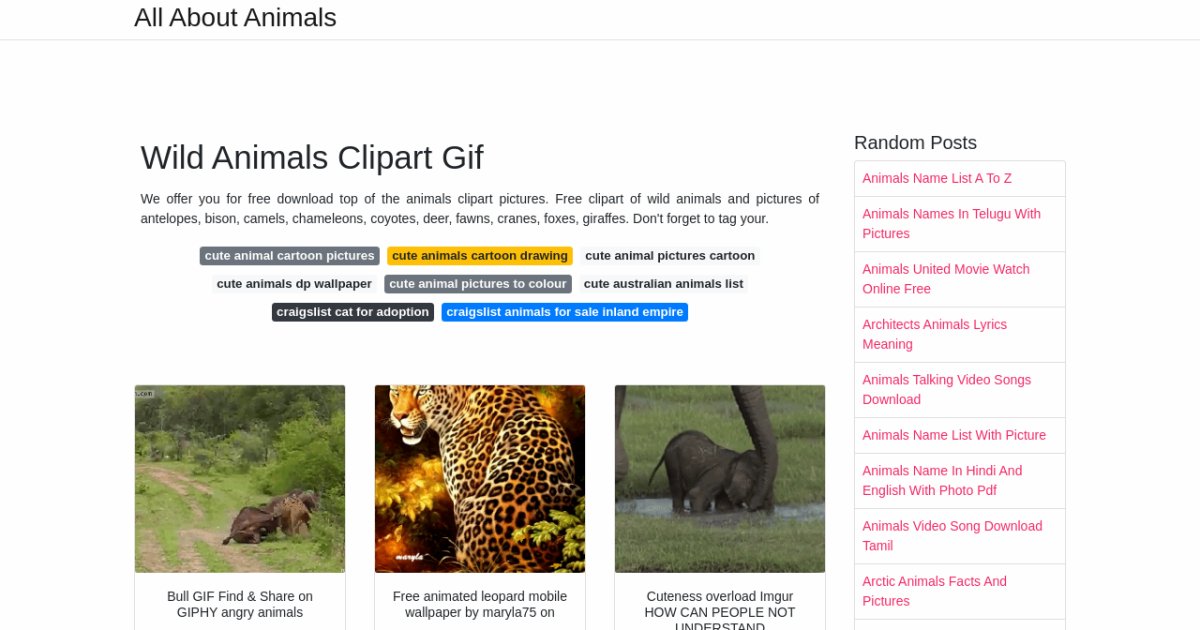At the top of the image, there is a black heading that reads "All About Animals." Below this is a thin gray line running horizontally across the image. Under the line, in black text, it states, "Wild Animals Clipboard Gift." Another line of black text reads, "We offer you a free download of top animal clipboard pictures. Free clipboards of wild animals and pictures of antelopes, bison, camels, chameleons, coyotes, deer, fawns, cranes, foxes, giraffes."

Further down, there's a directive: "Don't forget to tag your..." followed by several boxes with different captions. The first box is gray with white text that says, "Cute Animal Cartoon Pictures." The next box is yellow with black text, "Cute Animal Cartoon Drawings." Another black box reads, "Cute Animal Picture Cartoon." The subsequent boxes are as follows: "Cute Animal DP Wallpaper" (white text on black background), "Cute Animal Pictures to Color" (black text on a white and gray background), "Cute Australian Animals List" (white text on black background), "Craigslist Cat for Adoption" (black text on white background), "Craigslist Animals for Sale and Land Empire" (white text on blue background).

Following this is a section with three images. The first image appears to be of a lion and a tiger with the caption, "Bull, Gif, Find and Share on Giphy, Angry Animals." The second image is of a cheetah, captioned "Leopards Mobile Wallpaper by Marla75." The third image features a baby elephant with the text, "Cuteness Overload, Ignore. How can people not understand?"

Finally, there are several random posts in assorted colors, culminating in:
- A magenta box that says, "Animal Name List A to Z with Pictures"
- "Animals United Movie Watch Online"
- "Architects, Animal Lyrics Meaning"
- "Animals Talk and Video Songs"
- "Animal Names in Hindi and English with Photo PDF"
- "Animal Video Song Download"
- "All Take Animals."